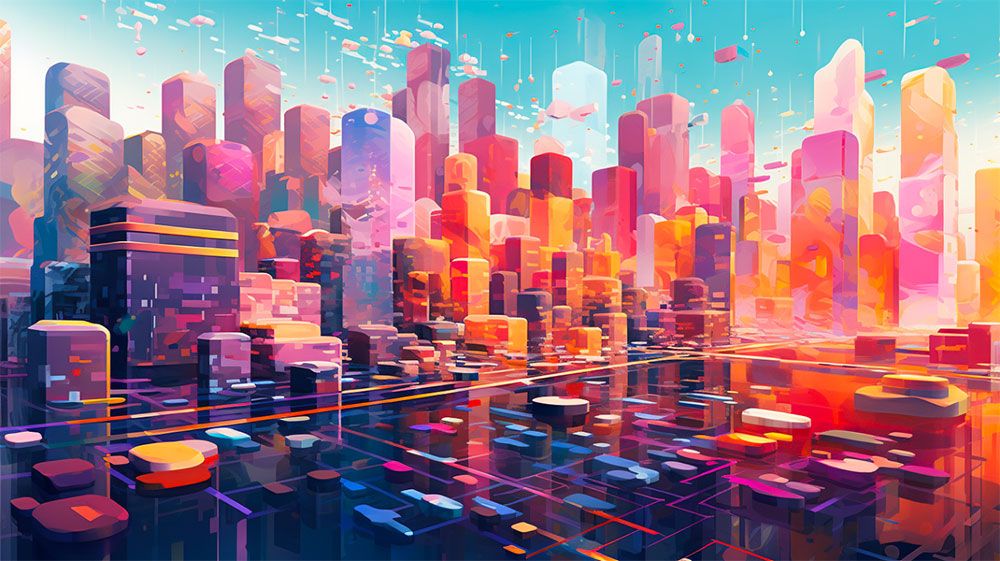This digital artwork represents a cityscape with a distinctive style, characterized by rounded and solid shapes that blur the details of individual buildings. The city skyline is fragmented into rounded, colorful elements with predominantly earthy and purple tones, giving the impression of a city abstractly merged with a natural landscape like the Grand Canyon. The bottom portion of the image features flatter, low-elevation structures or a vibrant ground surface filled with an array of varying shapes and colors, possibly representing a bustling foreground of streets or an ocean with vehicles and boats. Above the skyline, a vivid blue sky is punctuated by hanging rectangular and smaller shapes, adding a surreal dimension to the urban scene. The overall composition intertwines urban scenery with natural aesthetics, creating an intricate and colorful depiction of a modern metropolis.